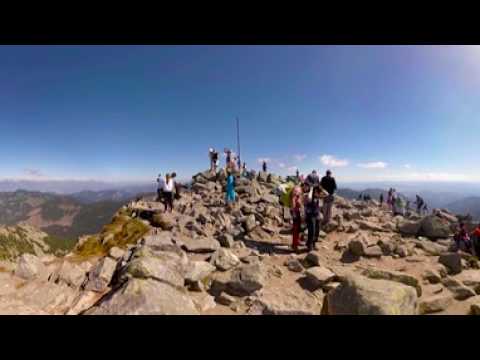This photograph captures a vivid scene atop a rocky mountain peak, where the terrain is predominantly composed of light gray and scattered rocks. A clear, azure sky stretches overhead, with a few white fluffy clouds visible along the horizon. The sun beams brightly from the top right corner, flooding the area with light. 

In the center of the image stands a tall, dark gray metal pole, marking the highest point of the peak. Surrounding this pole, a diverse group of hikers clad in gear and carrying backpacks either stand or move about, observing the panoramic views. These views encompass an array of distant mountains, which exhibit hues of green and gray. The lush greenery is visible below the rocky summit, providing a stark yet beautiful contrast to the ruggedness above.

People are dispersed across the mountaintop—some are clustered near the pole, enjoying the summit's pinnacle, while others are scattered closer to the vantage point of the camera. Everyone seems entranced by the scenic expanse around them, either gazing into the distance or contemplating their rocky surroundings.